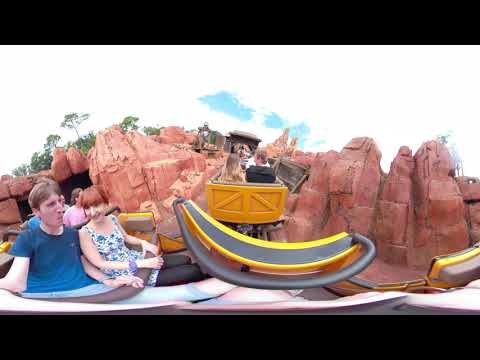The image is a panoramic, fisheye lens photo capturing a lively scene on a roller coaster ride, possibly at Disneyland. In the bottom left corner, a man is taking a selfie, wearing short blue denim jeans pulled above his knees and a short-sleeve blue shirt. Close beside him, holding on to the gray metal safety bar and brown padded bar, is a woman with red hair, smiling. She is dressed in a thin-strapped white top adorned with green and purple flower patterns, and black pants. Both are seated in a connected series of yellow carts with gray metal bars in front. The roller coaster is adorned with fake, cosmetic rocks on either side, creating a faux-stone environment. The ride appears to be curving, suggesting an upcoming uphill climb. Behind and in front of the couple, other riders in similar carts can also be seen, soaking in the thrilling experience. The sky is partly cloudy with patches of blue, and there are trees visible in the background, adding to the scenic amusement park atmosphere.